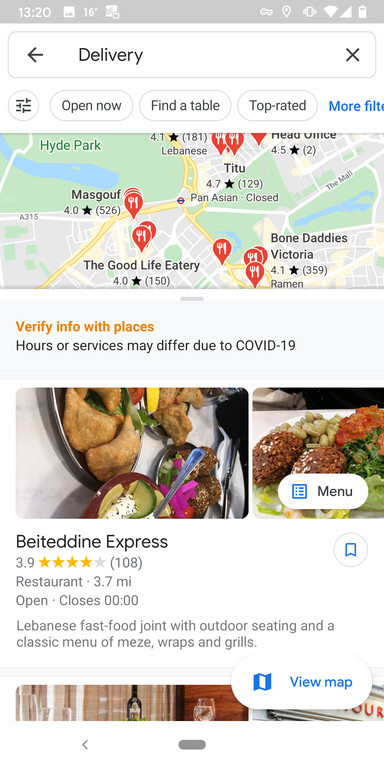**Descriptive Caption for Mobile Screenshot of Web Results:**

The image is a detailed screenshot from a mobile device displaying search results for "delivery." At the very top, a gray status bar shows common cell phone indicators: the left side displays the time in military format, 13:20, alongside several icons representing functionalities understood by the user, including a temperature icon reading 16°C. On the right side of the gray bar, standard icons for Wi-Fi signal strength and battery life are visible.

Just below the status bar, a search box appears with the word "delivery" typed in. The search box includes an option to return to the previous screen or clear the search term using an 'X' button.

Directly under the search box, the layout resembles Google Maps, featuring several oval-shaped filter options such as "Open now," "Find a table," "Top rated," and "More filters." To the left side of these options is an icon likely used for additional filtering or settings.

Beneath the filter options, a map highlights various eateries, some labeled with their names and Google star ratings. The interface includes a disclaimer reminding users to verify information since services may vary due to COVID-19.

Following the map, detailed information on specific restaurants is provided. Notably, there is a section for Bytadine Express, a Lebanese fast food restaurant. This restaurant has received 3.9 stars from 108 reviews, is located 3.7 miles from the user's current location, and has operating hours listed as open, closing at midnight. Descriptive text notes it offers outdoor seating and a classic menu comprising maize wraps and grills. Accompanying the description are images of Asian cuisine, with an option to access the full menu.

At the bottom, users can opt to view the map further, with a partial image suggesting the next restaurant in the search results.